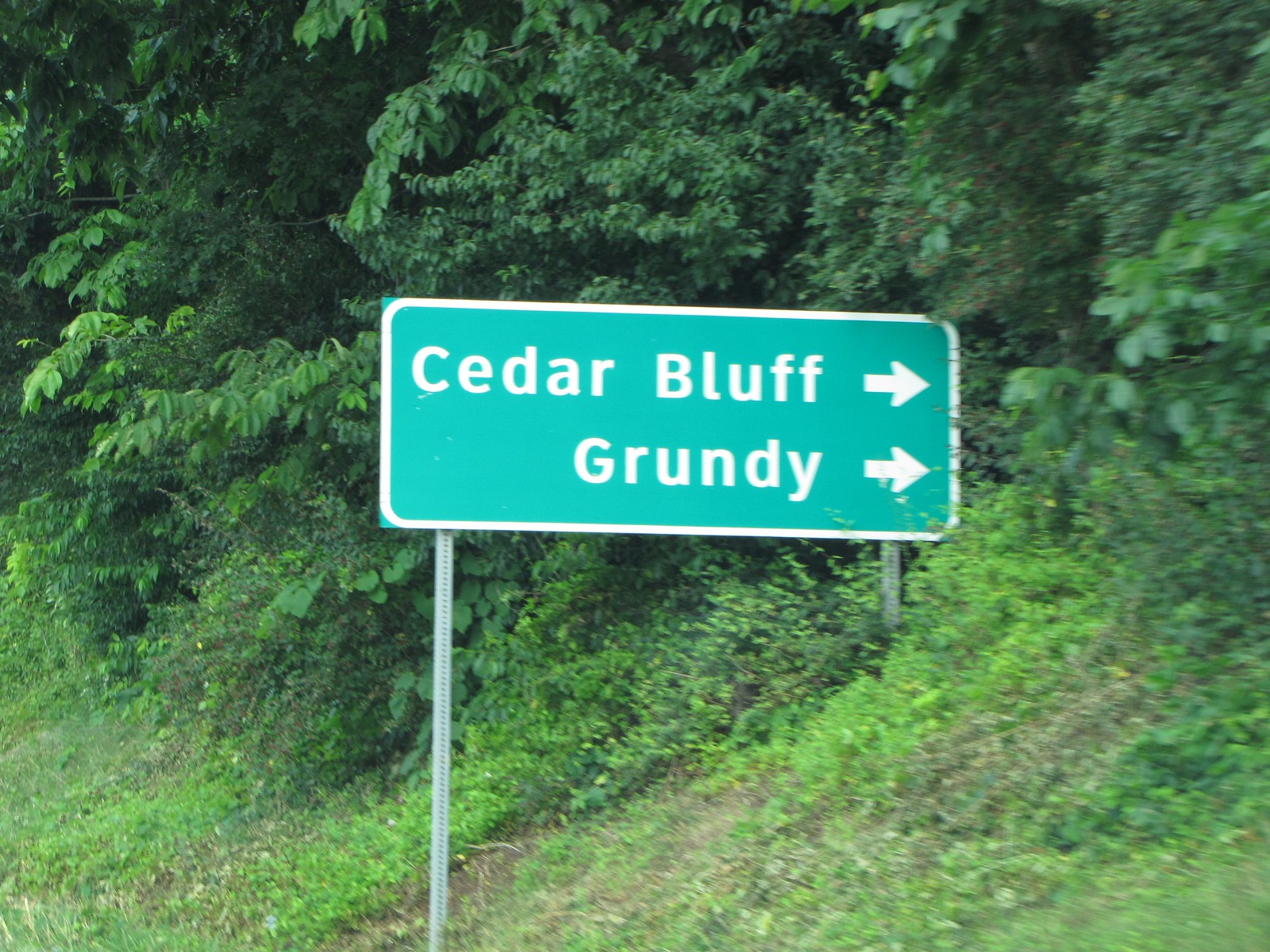A rectangular, light green street sign stands on the side of a road, its white-gray metal legs partially obscured by large, lush green bushes. The sign, which features white arrows pointing to the right, prominently displays the names "Cedar Bluff" and "Grundy." The vibrant, fluffy bushes cover the right leg of the sign, adding to the natural setting. Behind the sign, a dense array of leaves and foliage can be seen, with trees towering above, creating a verdant backdrop that envelops the entire street scene.